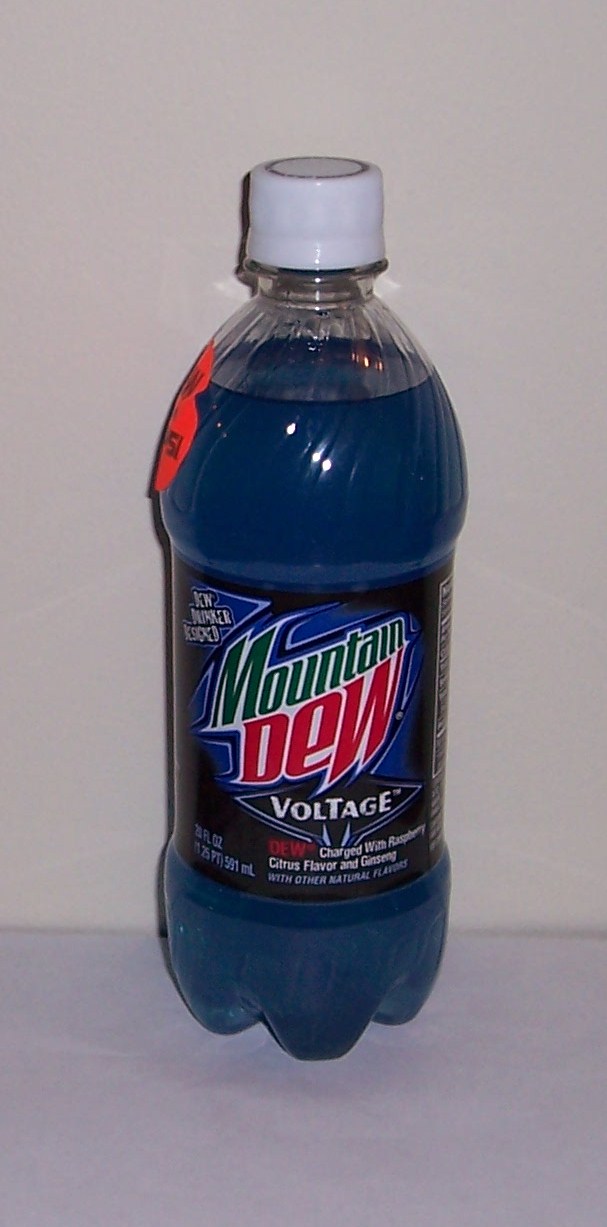This detailed indoor close-up photograph captures a 12-ounce bottle of Mountain Dew Voltage, a flavor characterized by its deep blue liquid. The bottle is plastic with a white cap and features a distinct black label. The label prominently displays the Mountain Dew logo, with "Mountain" in green and "Dew" right below it in capital letters. At the center, within a diamond shape, the word "Voltage" is visible, followed by fine print stating "charged with raspberry, citrus flavor, and ginseng with other natural flavors." An orange price sticker is noticeable towards the upper left side of the bottle, though its text is unreadable. The bottle sits on a gray table against a white wall, illuminated by bright lighting that includes the reflection of a flash near the upper part of the image. The drink's surface appears undisturbed, indicating the bottle hasn't been moved recently. The photograph is well-focused and well-lit, highlighting the contrast between the vibrant blue liquid and the stark white background.